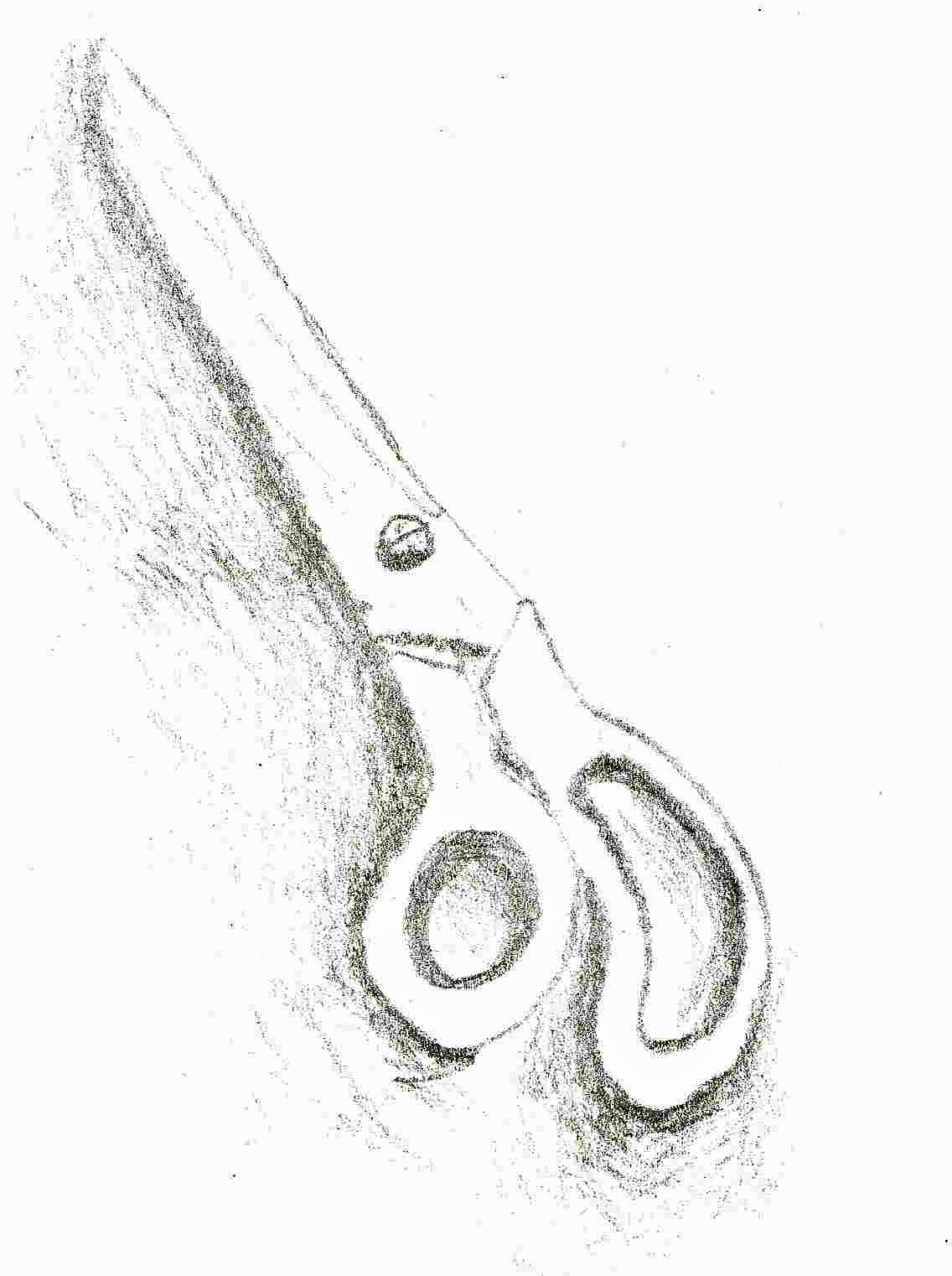This image features a detailed sketch of a pair of scissors, rendered in black and white against a white, lightly textured background, likely a piece of paper. The scissors themselves are depicted with intricate shading and black markings that accentuate their edges and surfaces, suggesting a drawn medium such as colored crayons or gray pencil. The scissor blades, facing towards the top left of the image, are connected by a distinctive slotted screw at their pivot, and they feature a white interior contrasting against their dark outlines. 

Each handle is uniquely shaped; the left handle is circular, while the right handle is more oval or bean-shaped. Both handles have faint gray shading inside, adding depth to the sketched depiction. The handles are positioned near the bottom of the image, with the blades extending upwards. A subtle shading on the surrounding surface further anchors the scissors to their illustrative space, emphasizing both the simplicity and meticulous detail of the drawing.